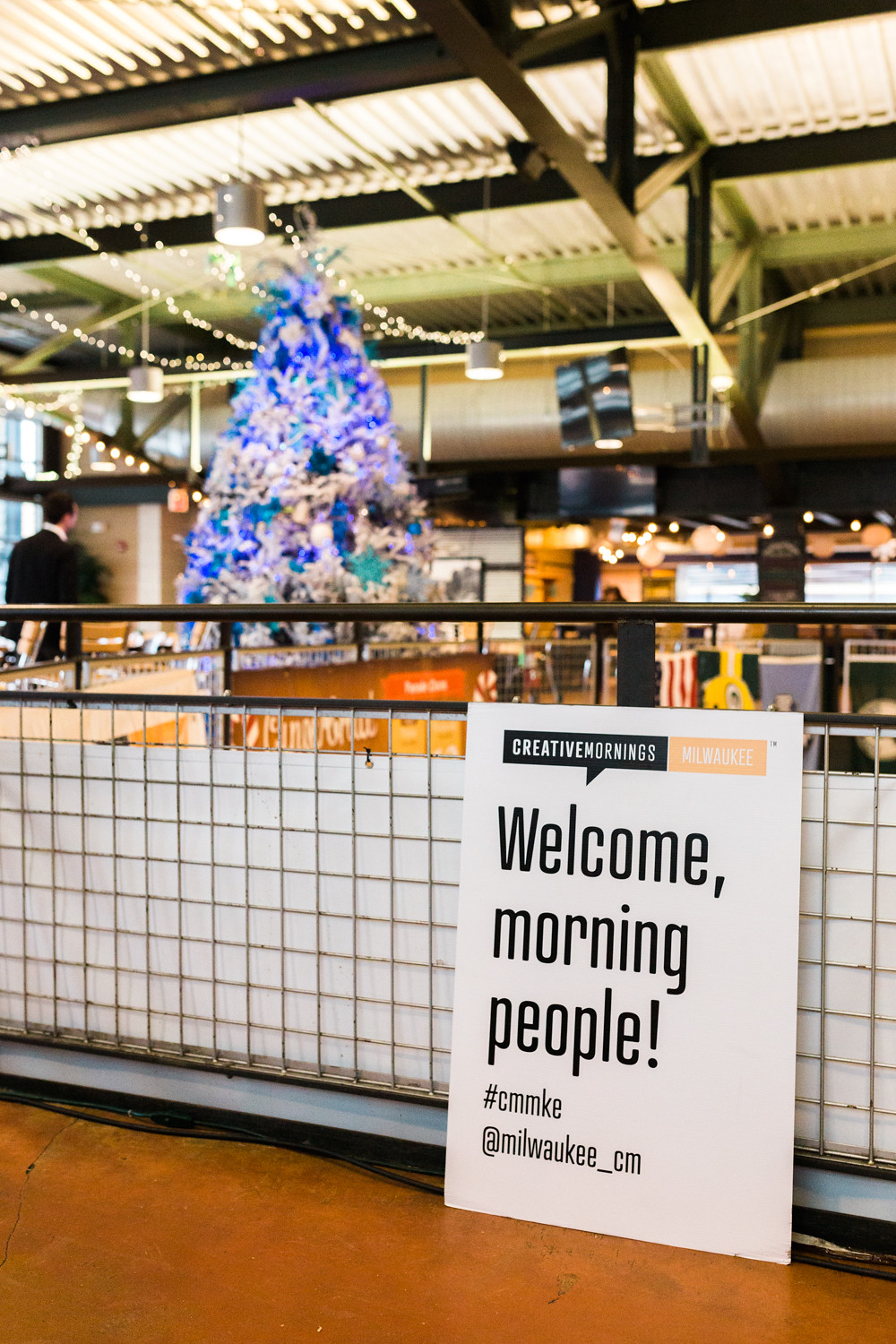This image captures a lively and festive scene in what appears to be an event space, possibly within a mall or restaurant setting. A prominently displayed white banner draped over a decorative metal railing reads "Creative Mornings, Milwaukee" and "Welcome morning people!" alongside hashtag "CMMKE" and social media handle "@Milwaukee_CM". Illuminating the background, a large Christmas tree adorned with a mix of purplish, blue, white, green, and other colorful ornaments and lights adds to the celebratory atmosphere. Above, white string lights are strung across a beautifully designed and patterned roof, contributing to the festive décor. The area sits on an upper floor, as evidenced by a railing overlooking a lower level with visible signboards for various shops or restaurants. To the left, a person in a black suit and white shirt with dark hair walks away from the camera towards the tree, adding a sense of motion and human presence to the scene. The overall architecture and lighting give the space a welcoming and creative vibe, perfectly suited for the event being celebrated.